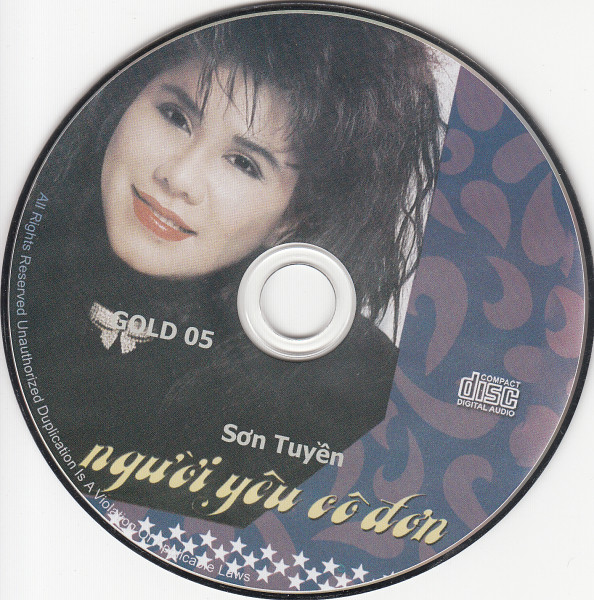The image features a compact disc with a black rim and an array of text around it stating, "All rights reserved, unauthorized duplication is a violation of applicable laws." The disc's design is dominated by a background blend of dark blue and deep purple hues, complemented by rows of light purple stars at the bottom. Central to the image is the CD itself, which showcases a smiling Asian woman with pale skin, adorned in a black outfit accompanied by a sparkling silver necklace. Her hair is black and appears a bit wild, styled messily but intentionally. She wears vivid red lipstick. The top part of the CD prominently displays the text "Gold 05," while the right section includes the phrase "Compact Disc Digital Audio." Additionally, the name "Song Tuyen" is displayed, followed by more text in what appears to be a foreign language, scripted in yellow font.